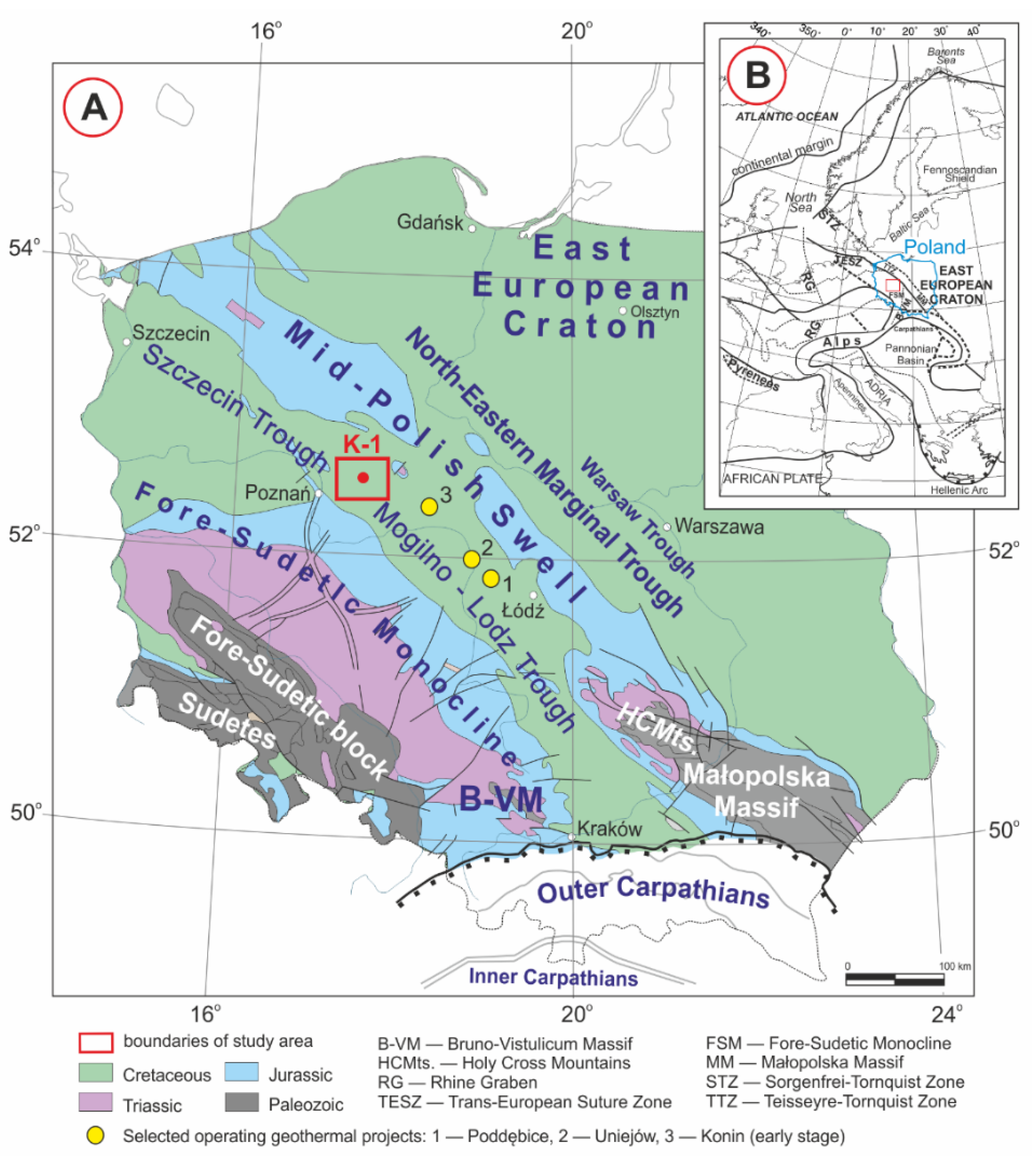This image depicts a detailed geological map of Poland, zoomed in on a section labeled "A," indicating the East European Craton, a vast plain area, and the Northeast Marginal Trough. An inset labeled "B" shows a broader view including the Atlantic Ocean and larger regional context. The map illustrates various topographical features such as the Warsaw Trough, Mid-Polish Swell with historical water presence, and other distinct formations like the Holy Cross Mountains (HCMTS) and the Malopolska Massif (MM).

The diagram is color-coded to signify different geological periods: green for the Cretaceous, blue for the Jurassic, purple for the Triassic, and dark gray for the Paleozoic eras. A key at the bottom helps interpret these colors along with other abbreviations like the Brunovistulicum Massif (BVM), Trans-European Suture Zone (TESZ), and the Tessera-Tornquist Zone (TTZ). Additionally, three yellow dots mark locations of ongoing geothermal projects: Poda Beach, Uniejów, and Konin in early stages. The map includes numerous cities and coordinates laid out in a grid format, providing an in-depth look at the region's geological diversity and history.